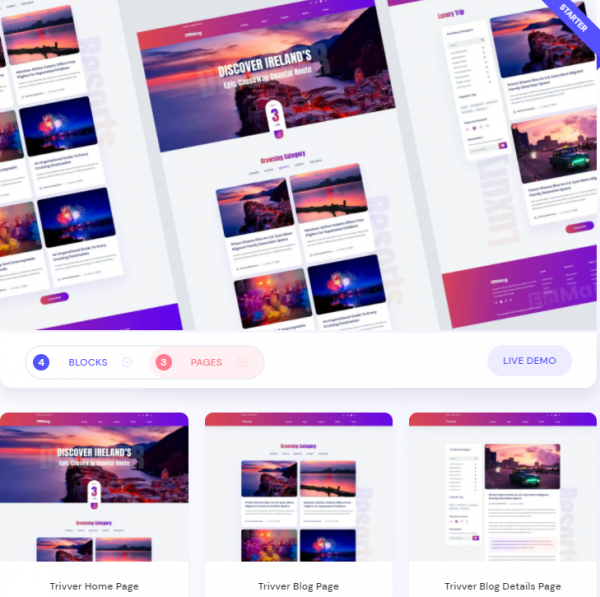The image serves as a promotional display for a website creation tool or service, potentially showcasing a proposed website design. It is divided into two sections. The larger section, occupying approximately two-thirds of the entire image, features a series of vertically-oriented, slanted website previews, predominantly hued in purple. These website previews depict scenic views reminiscent of Ireland.

At the center of this section, three slanted images are aligned together. The middle image prominently displays the text "DISCOVER IRELAND" in white, all-caps lettering, with some additional unreadable text beneath it. The scene within this central image portrays an island or a small village extending into the sea. Below these central images are four smaller landscape pictures.

The right section of the image seems to present an additional webpage, possibly containing a list. This section also features the same coastal image as the central one, accompanied by another landscape image. A purple banner reading "STARTER" in all caps is noticeable in this area.

At the bottom of the primary section, there are three distinct labels: "BLOCKS" on the far left, "PAGES" in the middle, and "LIVE DEMO" on the right. Beneath the slanted visuals, three more vertically-aligned images appear, but they are partially cropped and not fully visible.